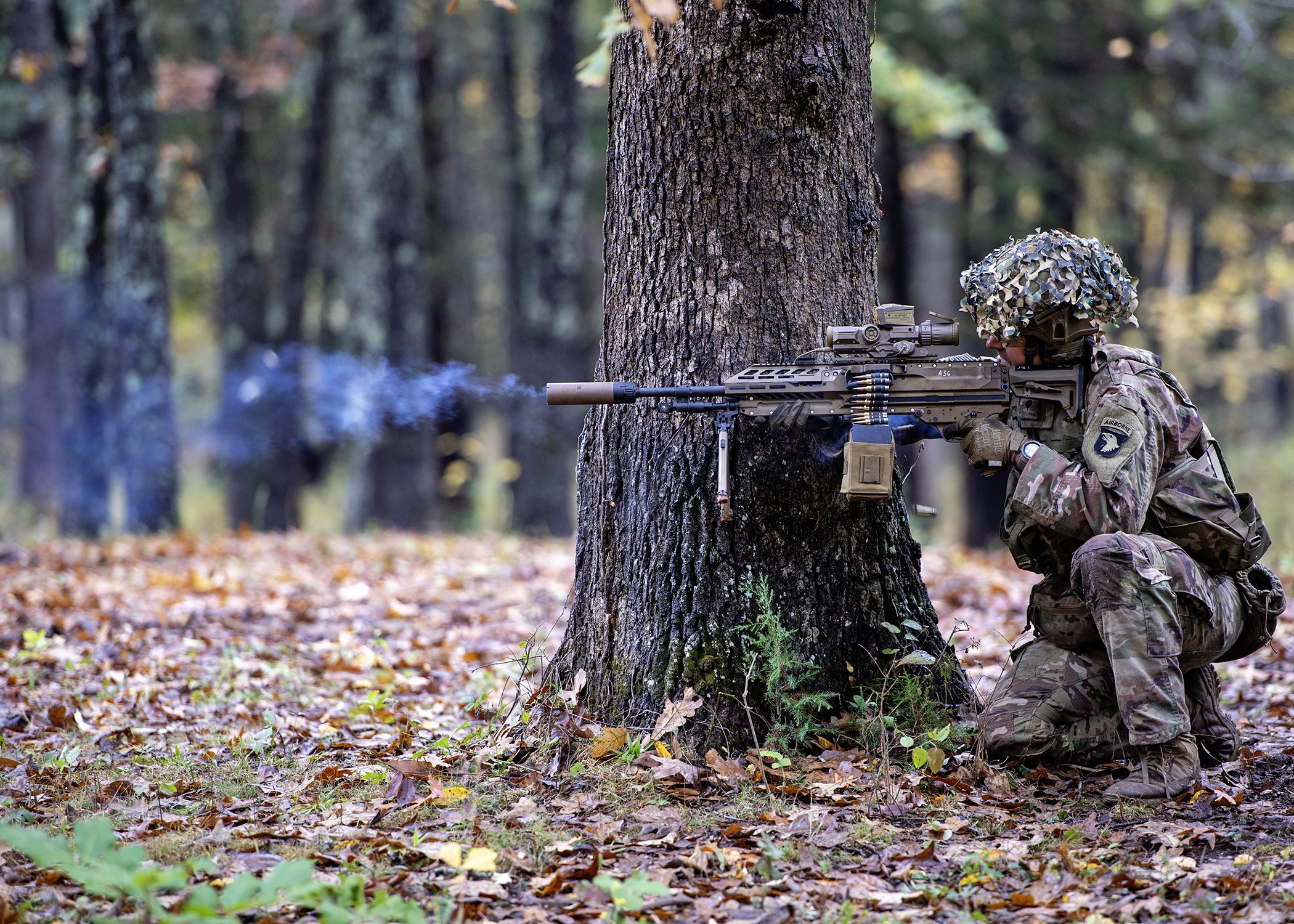In this detailed photograph, a man clad in military fatigues and a camouflage helmet, marked with an eagle emblem on his right shoulder and an air force patch, is captured in the midst of a military exercise in a forest setting. He is crouched behind the sturdy base of a tree, the ground beneath him adorned with a mixed palette of autumn leaves — some brown and dead, others vibrant and intact — depicting a fall scene. The soldier is intensely peering through the scope of a high-powered automatic assault rifle, from which wisps of smoke drift upwards, indicating a recent shot. His gear includes a matching camouflage watch and gloves, blending seamlessly with the surroundings. The dense woods stretch beyond him, featuring a mix of live plants and stark tree trunks, under the broad daylight filtering through the forest canopy.